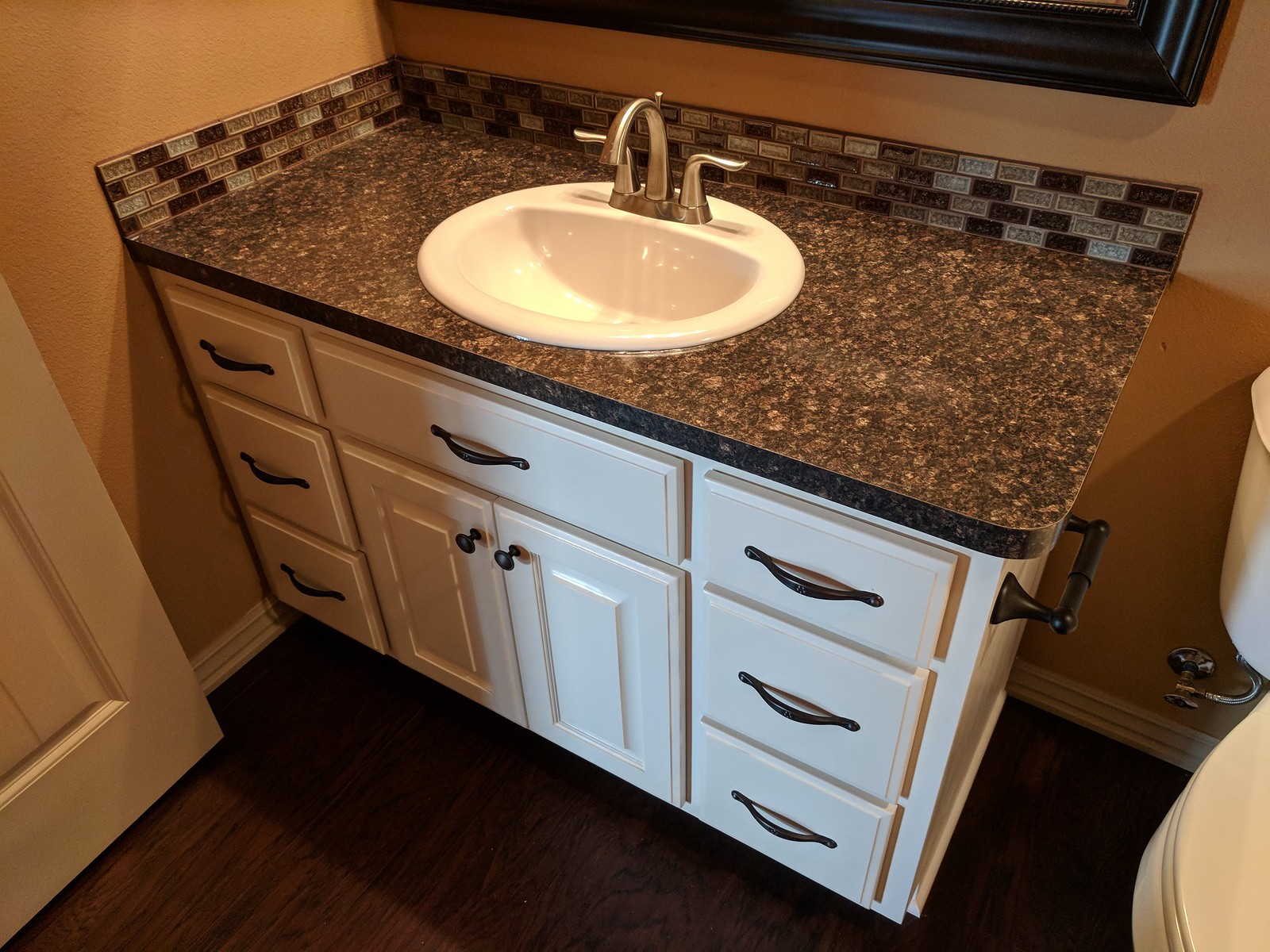This color photograph depicts a bathroom sink setup with striking clarity. The sink, which has a unique oval shape, is pristine white and features three taps: two on either side and a central curved tap. It is situated atop a countertop made of elegant black and greyish granite. The countertop is the centerpiece and is bordered at the rear by a narrow strip of small, square black and grey tiles, enhancing the sophisticated aesthetic.

Beneath the sink, a series of white cupboards and drawers provide ample storage. There are three sets of drawers flanking each side, while the central unit comprises a wide drawer above two spacious cupboards. All these drawers and cupboards are fitted with contrasting black handles or knobs, adding a modern touch to the overall design. 

The surrounding walls appear to be a warm brown hue, which complements the dark brownish flooring. Just above the sink, there is a dark frame which could either be a large photo frame or a mirror, suggesting a possibility that this space functions as a bathroom. On the left side of the image, a greyish cream door is partially visible, and on the right side, the round edge and cistern of a toilet can be seen, further indicating that this might indeed be a bathroom. The scene is illuminated by artificial lighting from above, casting a gentle glow over the entire setup, accentuating the clean and modern design of this bathroom.